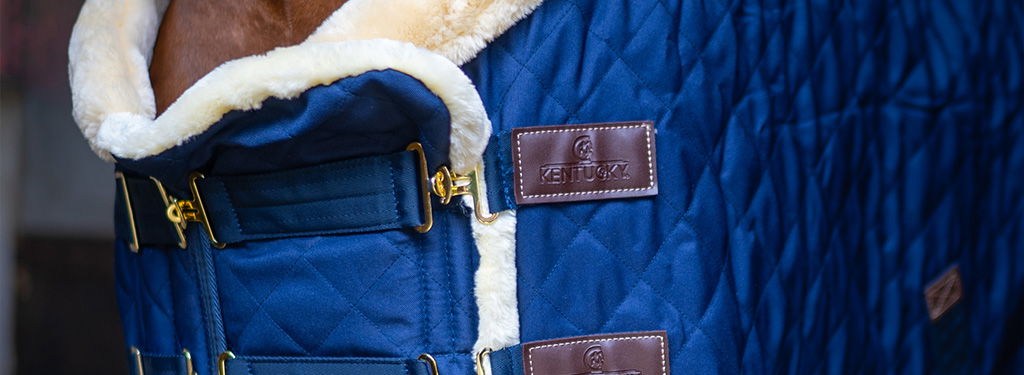The image is a long, horizontally rectangular photograph featuring a royal blue quilted horse blanket as the central focus. Visible at the top left is part of the horse's neck, which adds context to the blanket's purpose. The blanket is lined with soft, white Sherpa fabric, visible as a fluffy outline around its edges. The blanket is fastened with two buckles, each featuring golden brass fittings and blue straps that match the blanket's fabric. Attached to the buckle endings are brown leather patches, each engraved with the word "Kentucky" and an image of a horse, sewn on with visible white thread. The blue fabric has a diamond-stitched pattern, contributing to its quilted appearance.